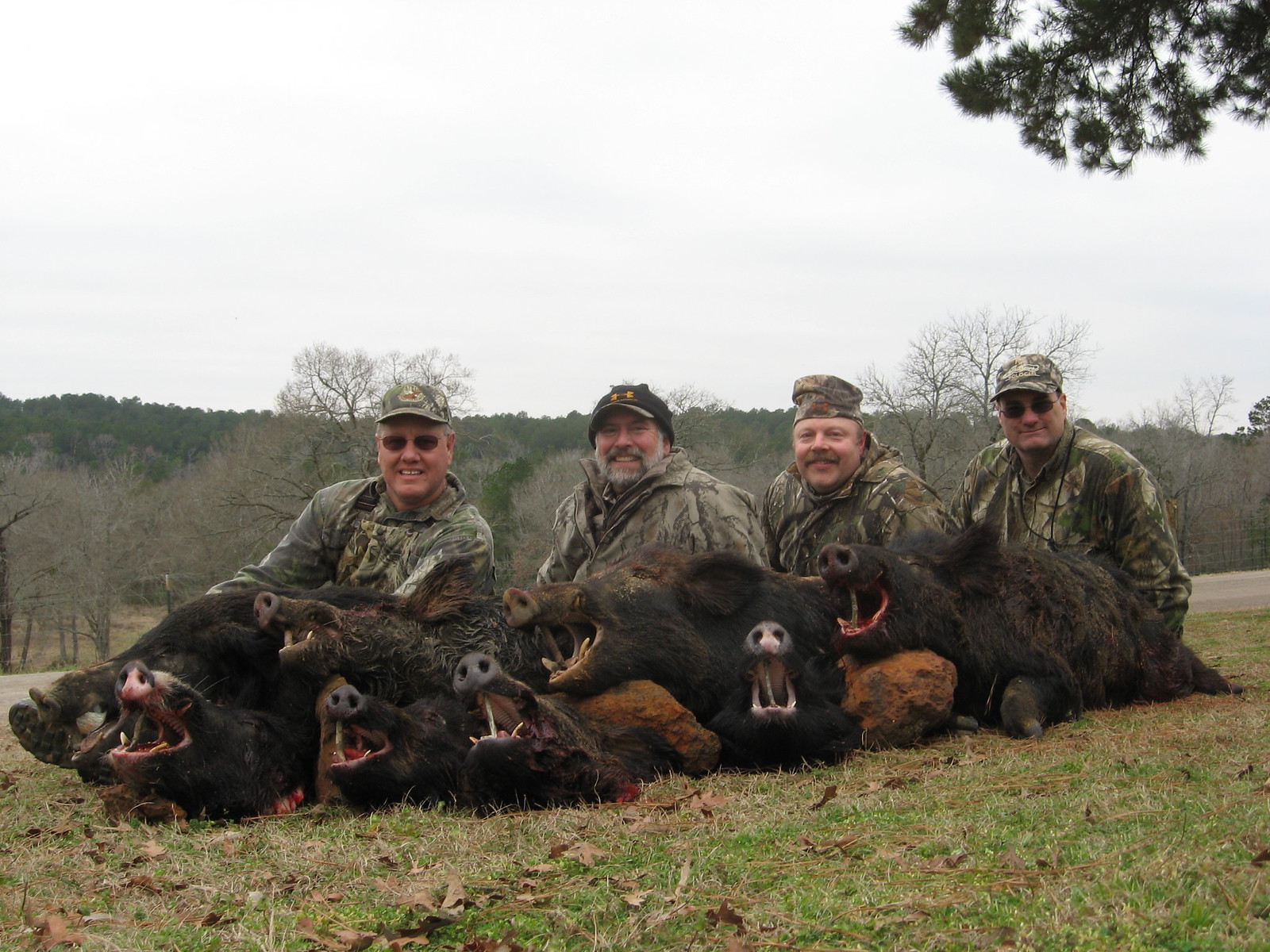This photograph features four hunters, dressed head-to-toe in camouflage gear including matching caps, sitting on a grassy hillside with trees in the distance. The skyline is hazy, suggesting an overcast day likely in a region resembling Kentucky, Tennessee, or Ohio. The men, identifiable as white with some sporting mustaches and others clean-shaven with sunglasses, pose proudly behind their game. Lying on the ground before them are seven wild boars, their dark bodies contrasting against the earthy background. Each boar has its mouth propped open with a stick, revealing prominent tusks—a grim showcase of their hunt. The hunters appear to be sitting amidst a mix of grass and fallen leaves, with more trees visible at the edge of the photograph, adding to the natural, rural setting.